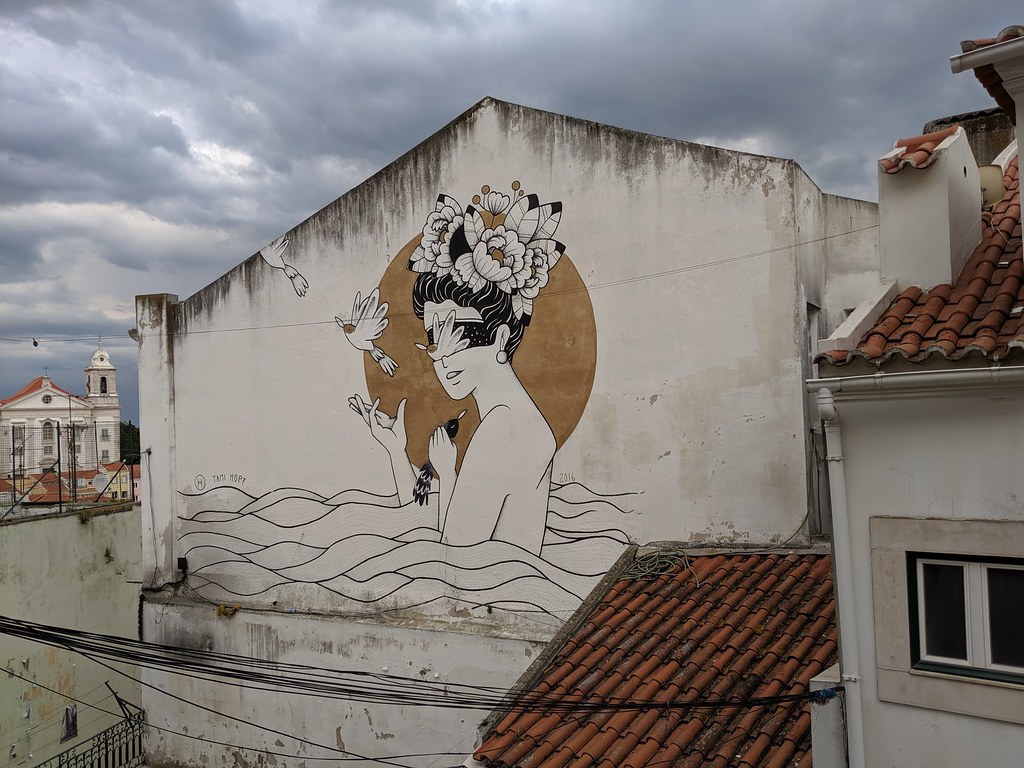The image captures the side of an older, white building in a predominantly concrete town, marked by gray streaks as if from coal dust or ash. This structure features a striking mural of a woman emerging from white-colored water. The woman, with black hair tied in a bun, wears a black mask over her eyes and has bright, large flowers and feathers of yellow, white, and black adorning her head. In a highly detailed scene, the woman releases white doves into the sky with her right hand while holding a single black feather in her left. The background of the mural shows a dim, orangish sun or moon. Surrounding this building, other white structures with terracotta roofs, evocative of European or possibly Victorian courthouse architecture, can be seen. One of these buildings, with a tall tower and many windows, possibly a church, stands prominently in the background under overcast and gray skies.